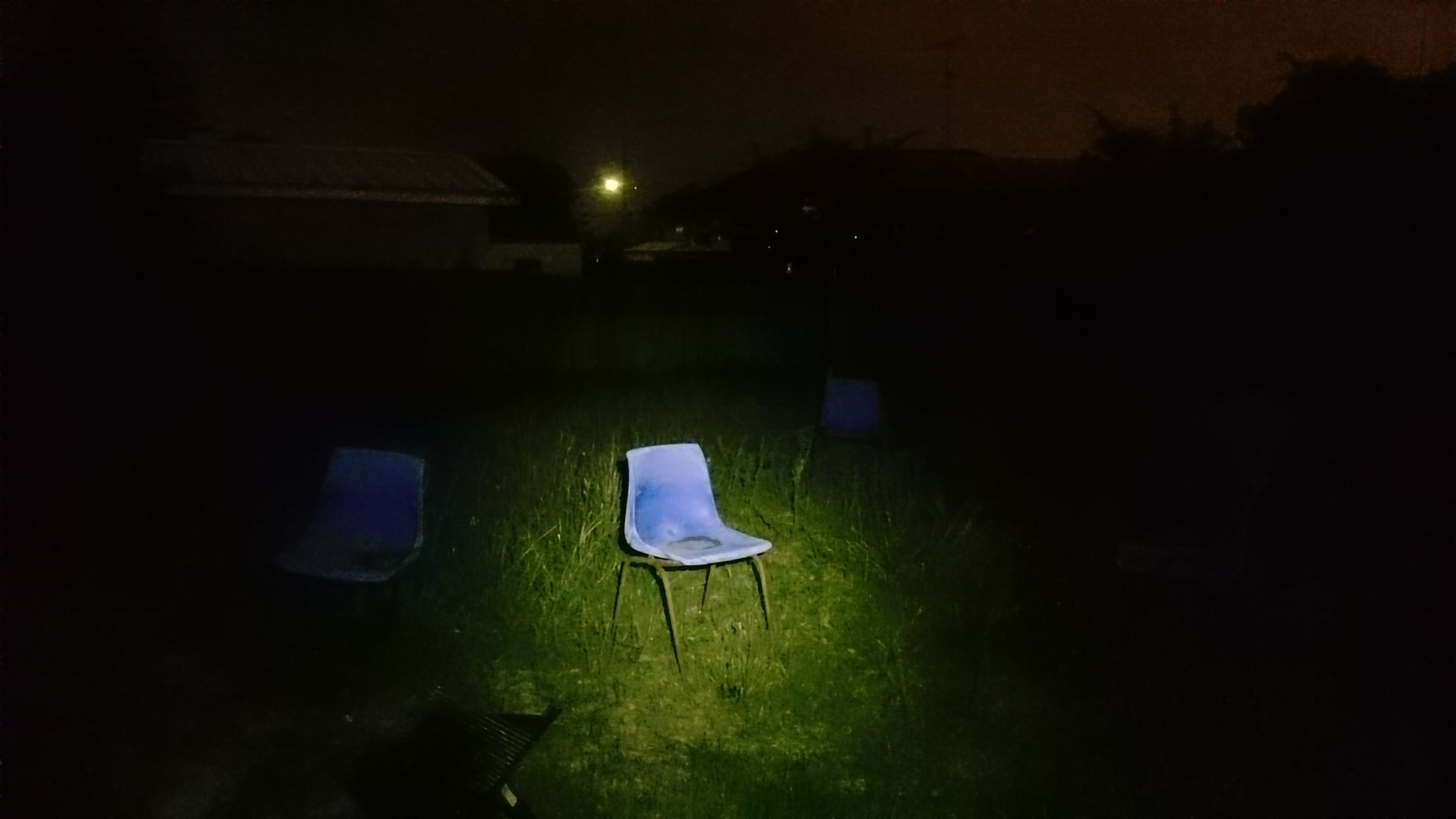In this nighttime photograph, an eerie atmosphere is created by the overwhelming darkness that envelops the scene, punctuated by spotlights. At the center, a solitary, old blue plastic chair with silver-toned legs rests on dark green grass, illuminated by a beam of light that shines down from above. The chair shows signs of wear, with potential puddles or bleached-out areas on its surface. The spotlight also reveals the texture of the grass around it, accentuating its presence.

To the left, the faint outline of another chair can be glimpsed, but it remains shrouded in darkness, blending into the black background that extends to the edges of the photograph. In the distant left background, there is a faintly visible structure resembling a standalone garage or barn, indistinct in the low light, with a bright light shining near it, possibly from a piece of equipment or a house. The horizon is barely perceptible, marked by a slight lightening of the sky and the shadowy silhouettes of trees. This contrast between the profound darkness and the isolated, lit elements adds a mysterious, almost haunting quality to the image.